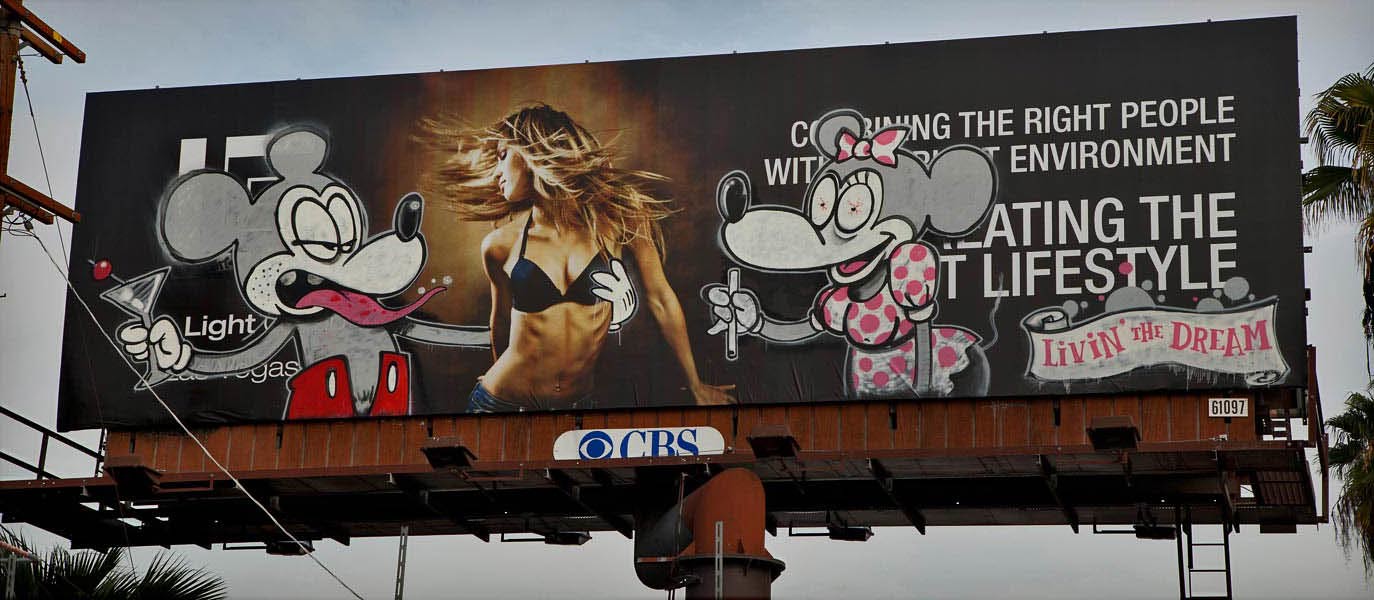In this photograph, a curious and risqué billboard stands out against a backdrop of gray sky and foliage at the bottom. Mounted on a rusty, brown metallic pole with visible ladders, the billboard has a black background and is partially obscured by graffiti. The central image features a woman with swirling hair, donned in a bikini top and jeans, facing forward but with her head turned dramatically to the left. To her left is a caricature of Mickey Mouse, sporting a bit of stubble, an unbuttoned pair of pants, and clutching a martini in his right hand. His left arm wraps around the woman as his tongue hangs out suggestively. On the right is a caricature of Minnie Mouse, dressed in her iconic white and pink polka dot dress and bow. She looks out of sorts, holding what appears to be a pipe, with tiny, dazed eyes.

The design is further accentuated by the CVS logo at the bottom, partially covered by graffiti. Behind Minnie, some of the original text is obscured but faintly readable, mentioning phrases like "the right people, the right environment" and ending with "the lifestyle, living the dream" in pink lettering. The image, while cleverly altered by graffiti artists, blends commercial elements with a satirical twist on beloved cartoon characters, casting them in a wildly uncharacteristic and provocative scenario.